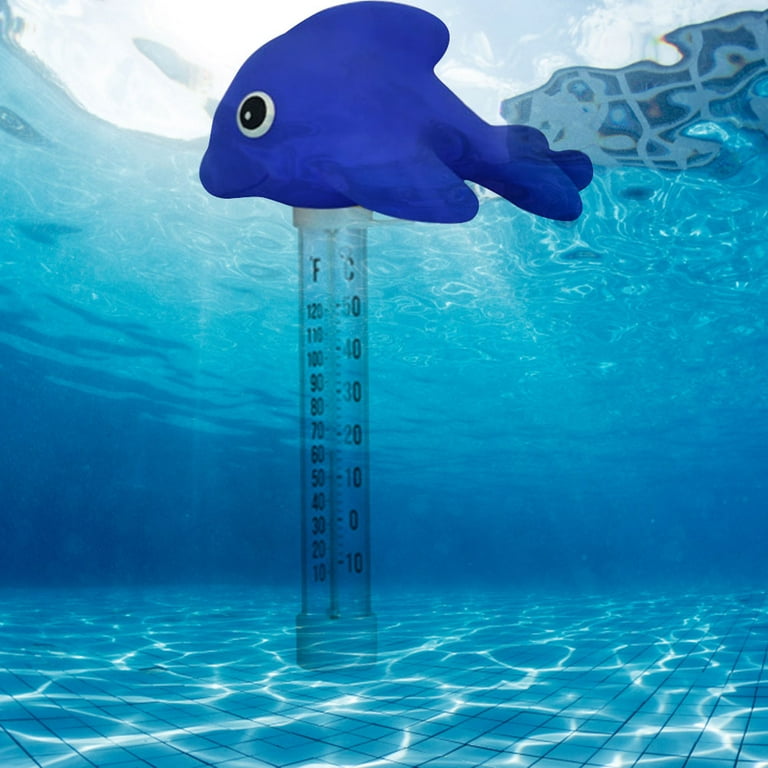The image depicts the bottom of a pool with pale turquoise water illuminated by sunlight. At the center of the scene stands an upright, see-through plastic thermometer, which features temperature scales in both Fahrenheit and Celsius: the Fahrenheit scale ranges from 120 to 10, while the Celsius scale ranges from 40 to negative 10. Perched atop the thermometer is a rubber toy fish, its side profile facing left. The fish is blue with a distinctive black eye, accented by a white ring and pupil, and a slight smile. The pool's tiles are visible, adding hints of dark blue, light blue, white, and gray to the scene.